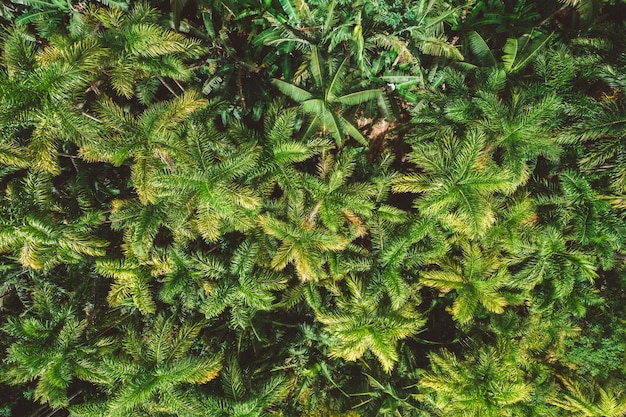An aerial photograph captures a dense, canopy-like carpet of palm trees, stretching as far as the eye can see, without any visible buildings or roads. The lush greenery dominates the image, creating a dark greenish background punctuated primarily by the overlapping fronds of the palms. While most of these fronds have a soft texture with dark green hues, some exhibit yellowed tips, adding a subtle variation in color. Shadows cast by the trees create a patchwork of darker areas, particularly noticeable in the upper middle, upper right corner, left bottom corner, and bottom middle of the photograph. Towards the top center, a different variety of palm tree stands out amidst the uniformity, adding to the intricate detail of the scene.